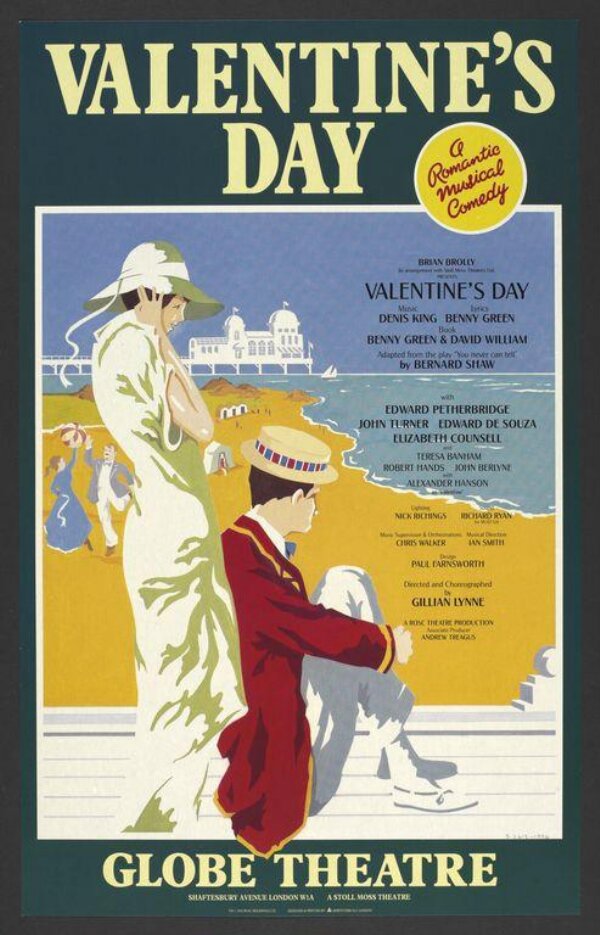The image is a scan of a poster promoting a theatrical show titled "Valentine's Day." The title, "Valentine's Day," is prominently displayed at the top in pale yellow letters against a dark blue background. To the right of the title is a small yellow circle with a white outline, containing the red text "a romantic musical comedy." 

Central to the poster is a detailed graphic of a woman in a sun hat, wearing a brown and white dress, standing on a white pier at a beach. In front of her sits a man holding his knees, dressed in a blue jacket and white pants with a light tan hat. The background features a serene beach scene with a blue sky and a body of water, alongside people playing ball and tents set up along the shore.

Below the illustration, several names appear in black text, including Dennis King, Benny Green, David William Bernard Shaw, Edward Putherbridge, John Turner, Edward D'Souza, and Elizabeth Council, suggesting they are involved in the show. At the bottom of the image, in pale yellow letters against the dark blue background, the location "Globe Theater" is indicated. The poster’s design effectively captures a sense of romance and musical comedy, inviting viewers to the performance.